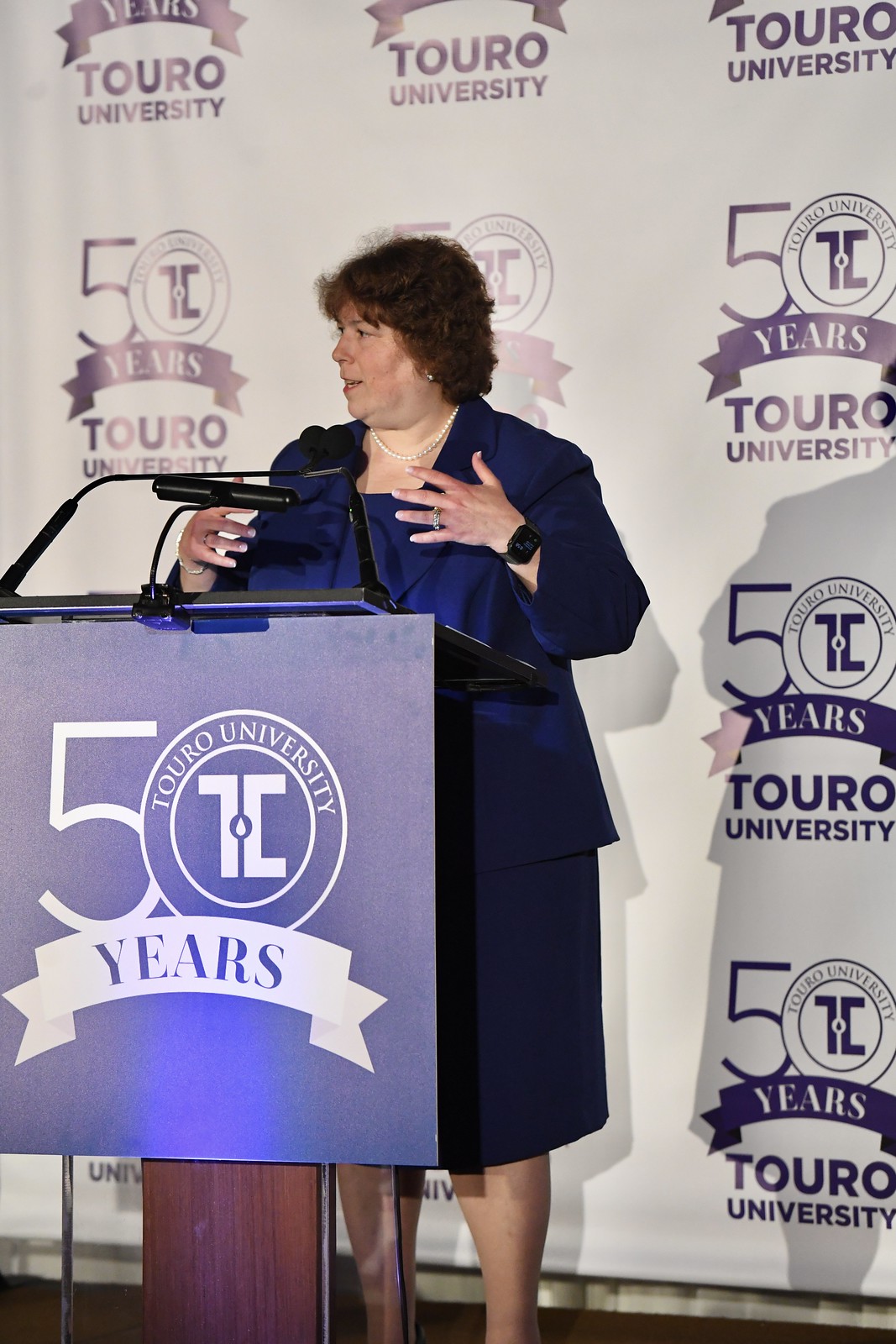In the image, an older woman, possibly in her early 50s, stands at a blue podium adorned with multiple microphones. She has short, curly brown hair and is attired in a professional, dark blue business suit that includes a vest, a modesty covering underneath, and a skirt. She also wears a black wristwatch and a wedding ring. Behind her, a prominent banner displays the text "50 Years Toro University" in blue and white. The banner features the Toro University logo, consisting of a stylized "T" and "C" with a white water drop in the center. This celebratory backdrop and her poised stance suggest she is speaking at a significant university event.